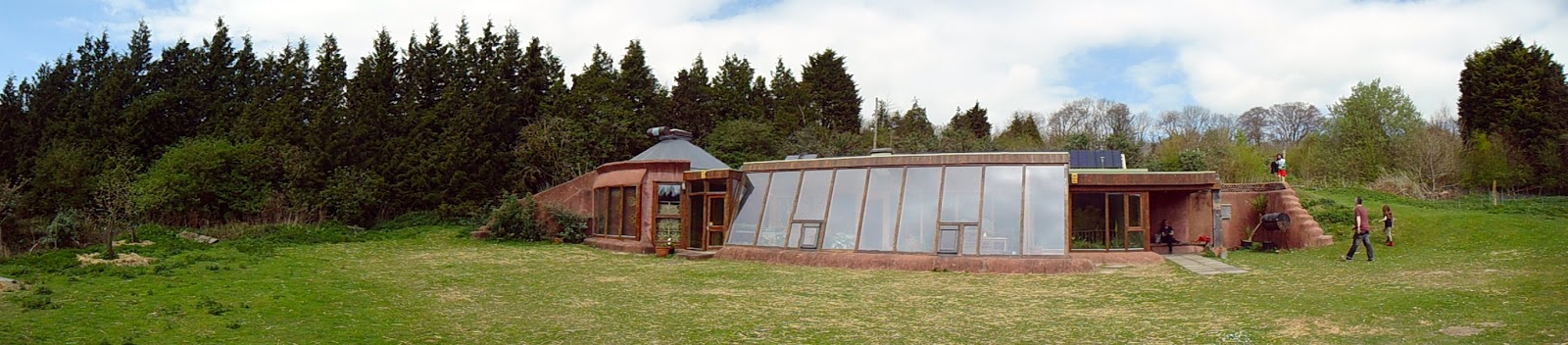The image depicts a long, rectangular, off-the-grid, self-built home, blending elements of a cabin and a standard house. This single-story, handmade structure, possibly constructed with red clay, features large, glass panel windows that angle backward, creating a greenhouse-like effect. Its surroundings consist of a grassy area with patches of light tan, dried grass, and it is nestled within a wooded area dominated by tall pine and deciduous trees. The sky above is blue with scattered white clouds, giving the scene a serene backdrop. The house has multiple wooden-framed doors on either side, with a distinctive round roof above one of them. There’s a hill behind the house, and people are visible in the image: some are walking on the hill, and one appears to be atop steps leading to the roof, while two others approach this individual. The panoramic, slightly warped perspective of the image offers an extended view, emphasizing the structure’s unique design and its integration with the natural landscape.